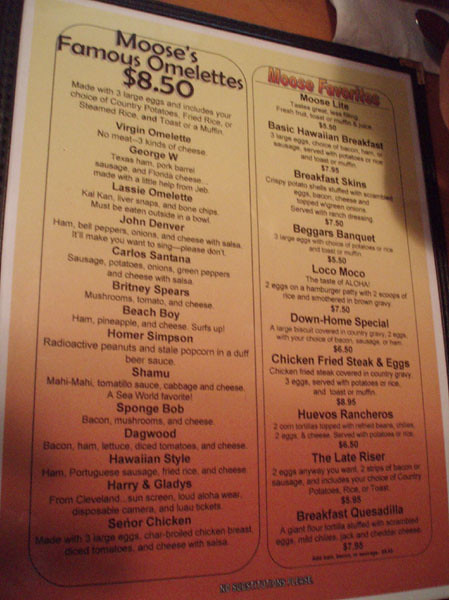In this indoor shot, we see a vibrant menu from a restaurant, prominently displayed against a yellow-orange backdrop. The menu details a variety of omelets, each with its own unique twist and playful names:

1. **Moose’s Stainless Omelet** - Priced at $8.50, this omelet is made with three large eggs and comes with your choice of country potatoes, fried rice, or steamed rice, accompanied by toast or a muffin.

2. **Virgin Omelet** - A meatless delight featuring three kinds of cheese.

3. **George W.** - This omelet includes Texas ham, pork barrel sausage, and Florida cheese, reportedly with a little help from Jeb.

4. **Lassie Omelet** - Contains Kai Kan, liver snaps, and bone chips, suggested to be eaten outside in a bowl.

5. **John Denver** - Made with ham, bell peppers, onions, and cheese, served with salsa. The menu humorously adds that it will make you want to sing, albeit with a plea not to do so.

6. **Carlos Santana** - Consists of sausage, potatoes, onions, green peppers, and cheese, also served with salsa.

7. **Britney Spears** - This option includes mushrooms, tomato, and cheese.

The whimsical descriptions add a charming and humorous touch to the overall vibrant aesthetic of the menu, making it as entertaining to read as it is appetizing.